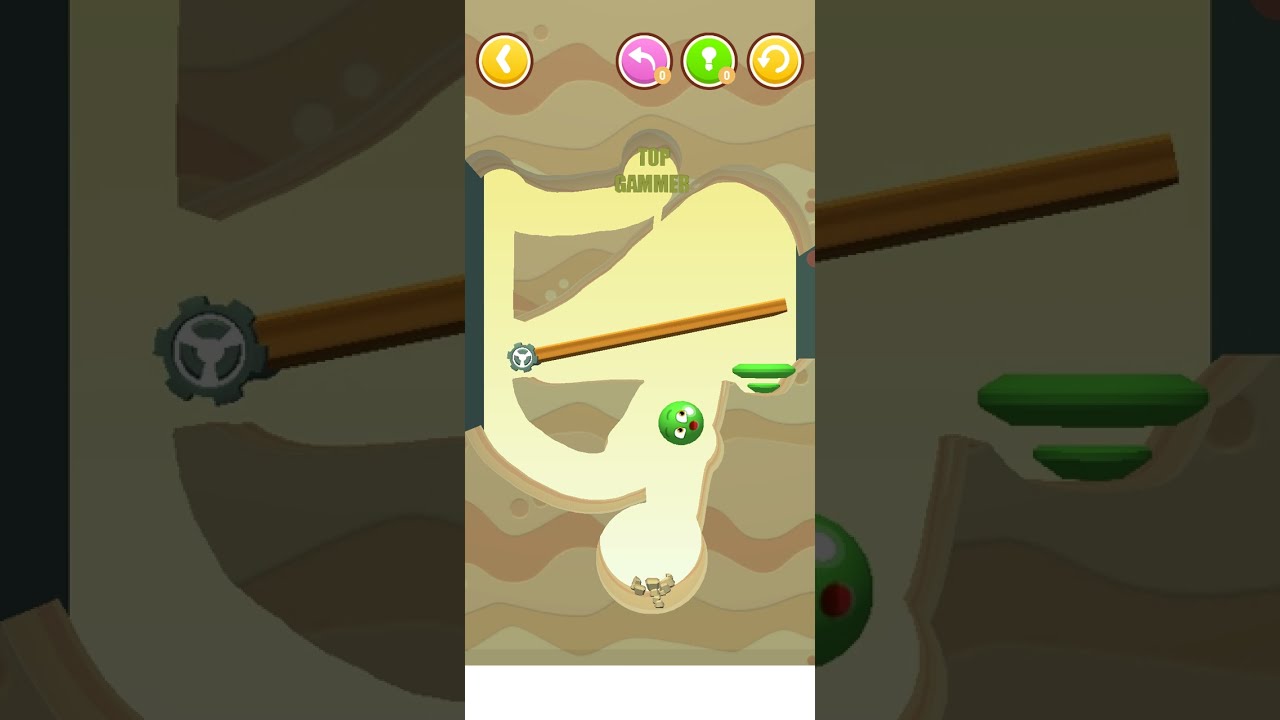The image appears to be a screenshot of a mobile video game, displayed within a vertical rectangle against a darker, zoomed-in background of the same scene. The game depicts a cartoon-style underground excavation area, showcased in a cross-section of dirt featuring a network of tunnels. Centrally, there's a green, ball-shaped character with eyes, a red mouth, and black eyebrows, resembling a green watermelon. This character is situated near a lever made of a wooden stick attached to a gray gear. At the top of the vertical game display, four buttons are aligned: an orange circle with a left-pointing arrow, a pink circle with another left-pointing arrow, a green circle with an exclamation mark, and a yellow circle with a refresh symbol. Below these buttons, the text "Top Gamer" (possibly misspelled as "Top Gammer") is written in green font, integrated into the earthy background that simulates various shades of brown and clay.